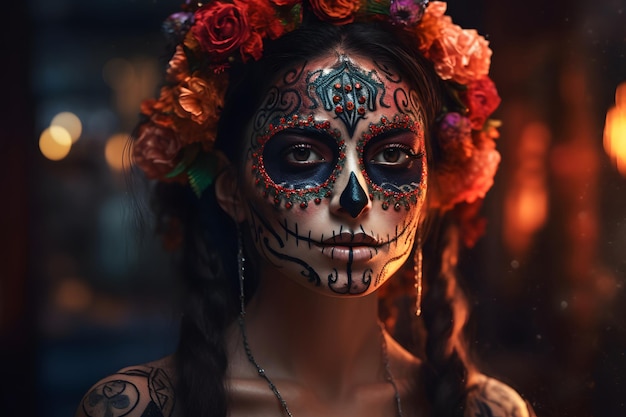This is a detailed photograph of a woman dressed for the Mexican Dia de los Muertos celebration, facing the camera with a calm expression. From the shoulders up, she is adorned with a large, vibrant flower crown in shades of orange, red, and purple. Her long brown hair is neatly styled in two pigtail braids. Her entire face is elaborately painted to mimic the traditional skull makeup associated with the holiday. Her forehead features a beautiful design encrusted with red diamond-like pieces and intricate green-black lines. The eye sockets are emphasized with navy blue paint, surrounded by a lacy red detailing and beads that create a hollowed, skull-like appearance. A black spot is painted on the tip of her nose. Her lips and cheeks display black lines that simulate a sewn-together mouth, complete with a delicate crisscross pattern extending into intricate swirls and curls. The dimly lit, blurred nighttime background enhances the striking contrast of her detailed face paint.